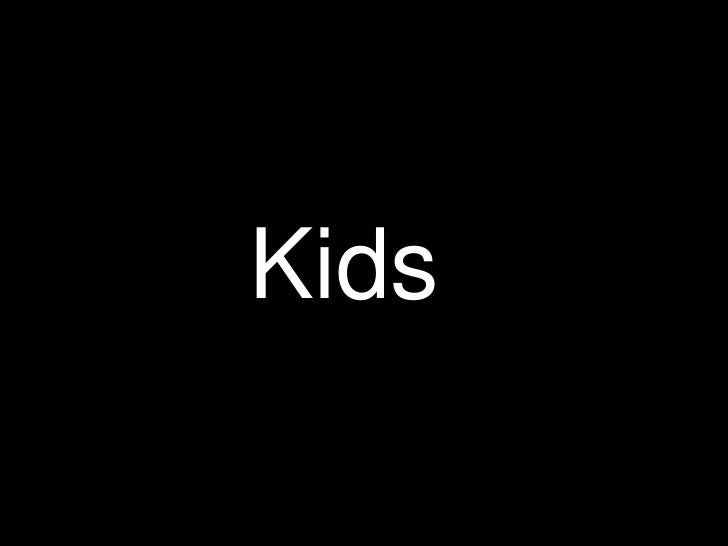The image presents a simple, all-black background with the word "kids" in the center, created using white text. The text is organized with a capital "K" followed by lowercase "i," "d," and "s," forming the word "kids." The font used is rigid with many straight lines, except for the letters "d" and "s," which incorporate some curves but remain simple and unornate. Notably, the dot above the "i" is a square. While the text is primarily centered, it appears slightly off to the top left. There are no other elements or distractions in the image—it is just the word "kids" on a stark black canvas.